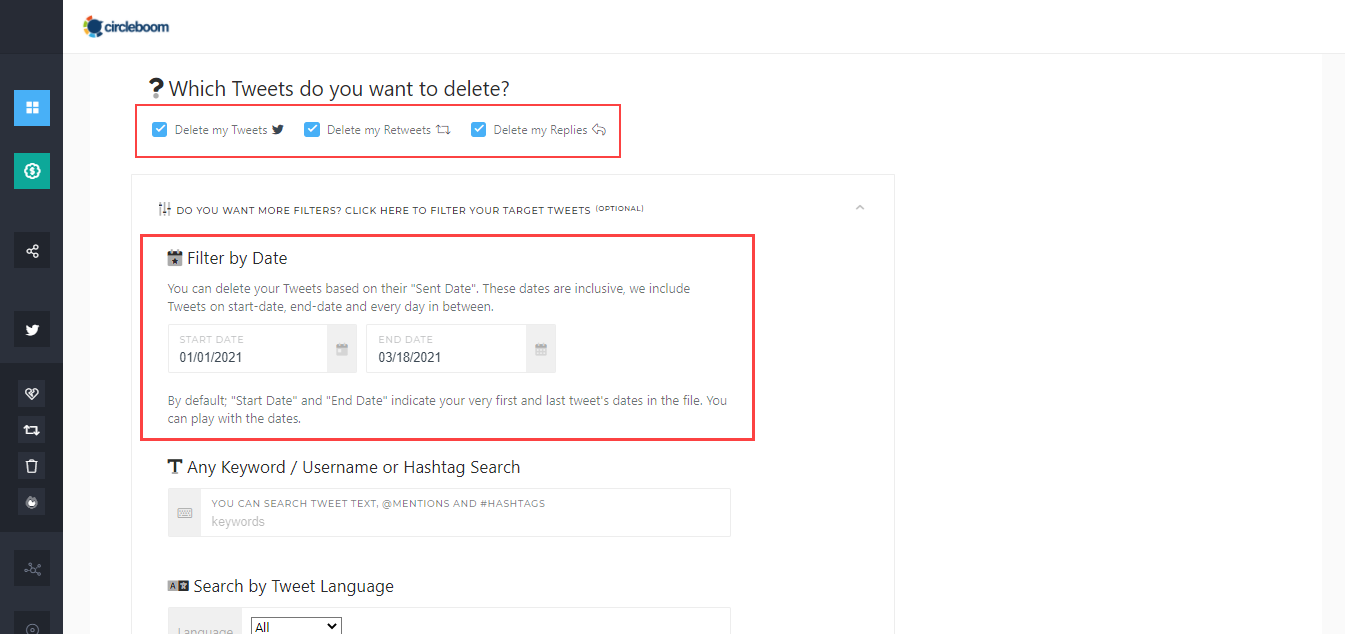On the left side of the image, there is a grey section. Adjacent to it, a prominent blue square displays the Microsoft Windows logo alongside an eye icon. Further to the right are various interactive buttons, starting with a "share" button, followed by a Twitter button, a heart icon, an arrow icon, and a cup icon. The image background features a muted grey tone.

Central to the image is a circular shape with a "boom" effect and a question mark next to it, posing the question, "Which tweets do you want to delete?" Below that, there is a tag that reads, "Want more filters?" with a clickable option to filter tweets. An optional red border highlights the section where users can filter tweets by their sent date. The filter instructs users that they can delete tweets within a particular date range. 

Example date selections show: 
- "Start date: 01/01/2021 - End date: 03/18/2021". 
By default, the start and end date fields indicate the user's first and most recent tweets.

Users are also provided options for advanced search criteria, including:
- Keywords/Usernames
- Integer values
- Hashtags
- Tweet text
- Mentions
- Tweet language

A drop-down menu is available for further filtering options, delineated by horizontal lines against a predominantly white background.